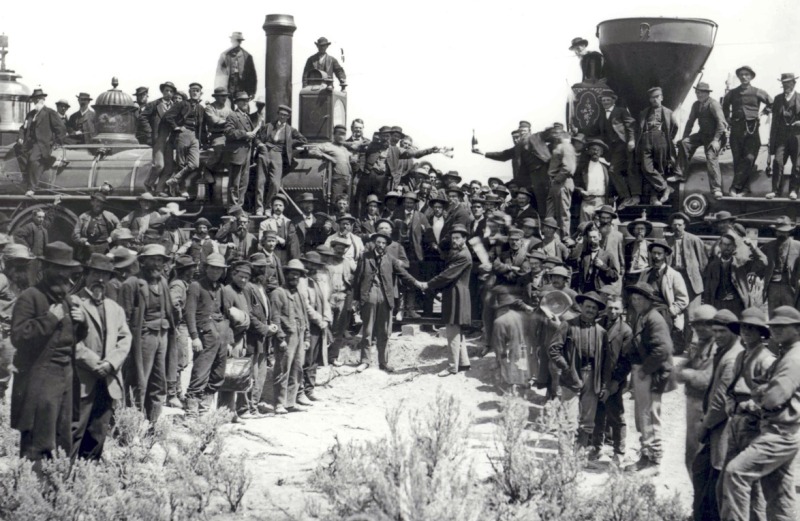This is an old black-and-white photograph, possibly from the late 1800s or early 1900s, capturing a celebratory moment in history. The image depicts a large group of men, many of whom are standing on the ground in rows and atop two locomotive engines positioned face-to-face on the same track. This suggests a celebration of the completion of a railroad track where construction teams, working from two directions, have finally met and connected the tracks. In the center of the image, two men can be seen shaking hands, symbolizing an agreement or union. The men are formally dressed, with some holding alcohol bottles and glassware, indicating a toast to mark the event. The setting appears to be a semi-desert arid area, with sand and scruffy bushes on the ground. The photograph, with both clear and blurry faces, captures the significance and jubilation of this monumental occasion.